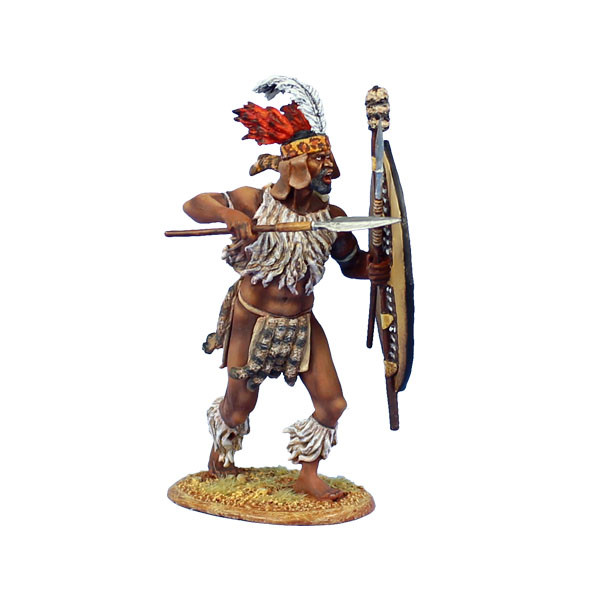The image depicts a highly detailed, colorful figurine of a fierce, dark-skinned male warrior, possibly of African or Aztec origin. The warrior stands on a round, earthy pedestal, hinting at a scene of battle or ceremonial importance. He is adorned in traditional garb with a golden headband that features a striking arrangement of red and white feathers, along with a striped grey and yellowish tail extending behind. His facial expression is one of intense anger, mouth open as if in a yell, and he has a beard and mustache. In his right hand, he wields a spear, while his left hand holds a wooden shield adorned with a fuzzy black and tan top, and a knife. His arms and forearms are decorated with tribal art.

The warrior's body is partially covered; a white feather chestplate shields his upper torso and similar white, frilly fabric flutters around his calves. His lower body is modestly covered by a loincloth with animal tails draping in front and back, leaving much of his muscular thighs visible. His right leg is bent, appearing to step forward, conveying a dynamic posture as if ready to strike or move swiftly. The figurine’s detailed craftsmanship suggests it could be a carefully crafted statue, a game piece, or a collectible model, notable for its vivid colors and emotive depiction.